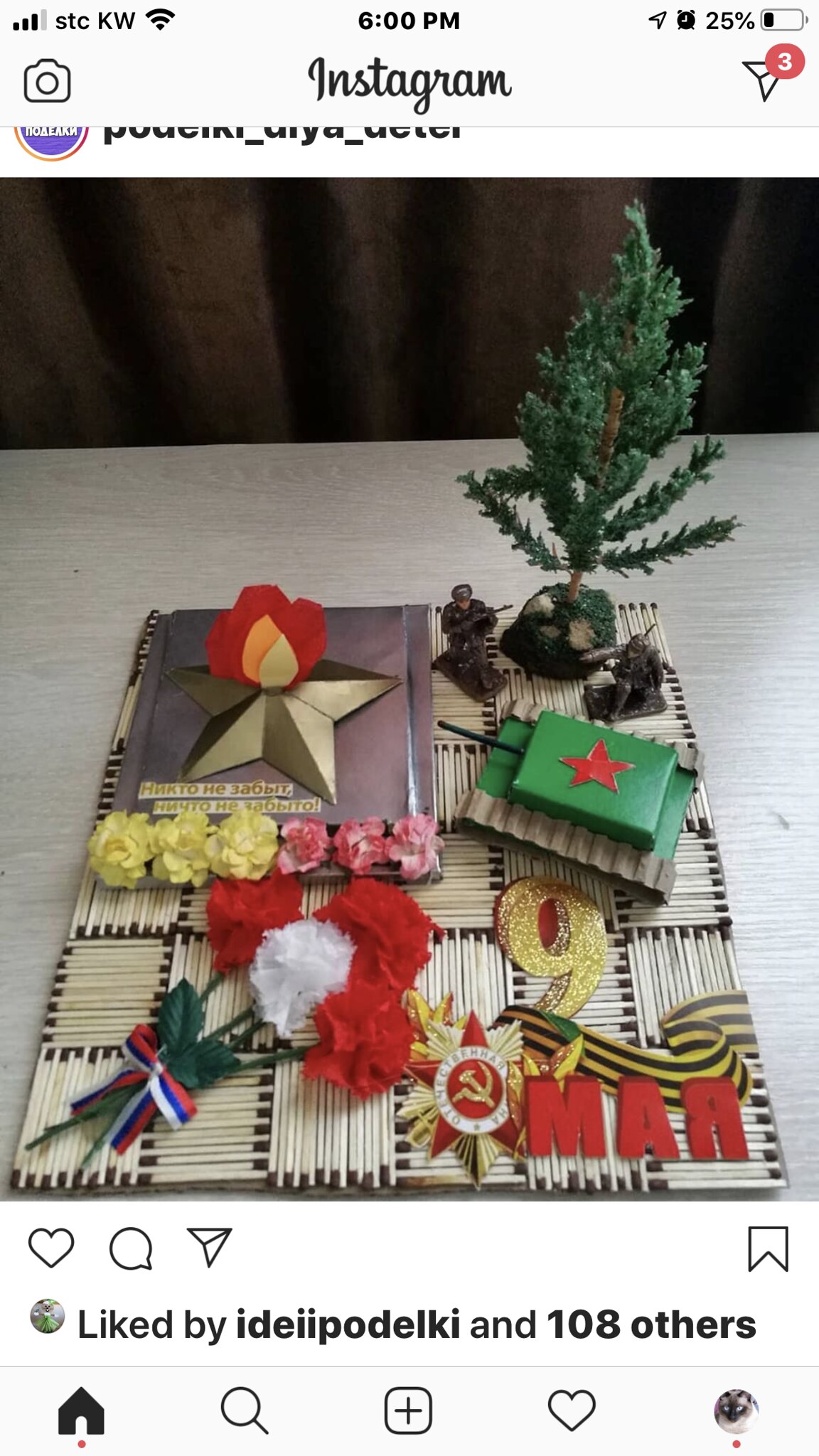The image is a detailed screenshot of an Instagram post captured from a mobile phone at 6 p.m., showing a 25% battery level and various standard screen indicators. The Instagram interface features the usual elements: the cursive "Instagram" logo at the top center, a camera icon to the left, a notification icon with a red circle indicating three notifications to the right, and an arrow pointing up to the top right. The handle of the Instagram account is mostly cropped out, but a purple avatar is partially visible in the top left corner.

The photograph within the Instagram post displays a top-down view of a festive Christmas-themed table arrangement. Central to the image is a small green Christmas tree with a brown base, possibly accompanied by tiny army figurines. Below the tree is a bright green notebook adorned with a red star. Adjacent to this notebook is the number nine, decorated with gold sparkles. Also present is a red circular emblem featuring a sickle and hammer, reminiscent of Soviet iconography, with the letters "M-A-R" to its right.

To the bottom left of the table display, there is a bouquet of artificial flowers tied with a bow in red, blue, and white, resembling the Russian flag. This bouquet comprises three red flowers and one white flower. Above it are six additional flowers: three yellow and three pink. A golden star with a small red circular object on top is also part of the arrangement. The background reveals black curtains at the upper section of the image.

At the bottom of the Instagram photograph, standard icons for liking, commenting, and subscribing are visible, alongside a bookmark icon. It says "Liked by IDI Pod Eelke and 108 others" in black text beneath the image. The Instagram toolbar is also displayed at the bottom, featuring icons from left to right: home, search, post, like, and an avatar within a circle, all set against a white background.